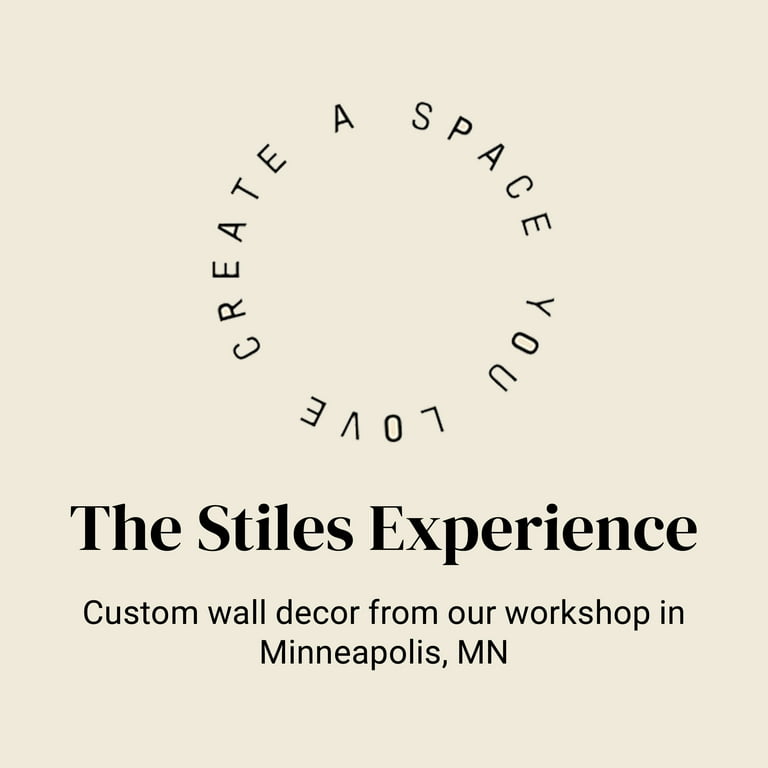Set against an ivory, pinkish-white background, this minimalist advertisement features elegantly simple black text. At the top, a circular formation reads "Create a Space You Love," with the center of the circle left blank. Below this, in bold letters, it states "The Styles Experience." Further down, smaller black text offers more detail: "Custom Wall Decor from our workshop in Minneapolis, Minnesota." This ad is purely text-based with no photographic elements, focusing solely on delivering its message with clarity and elegance.